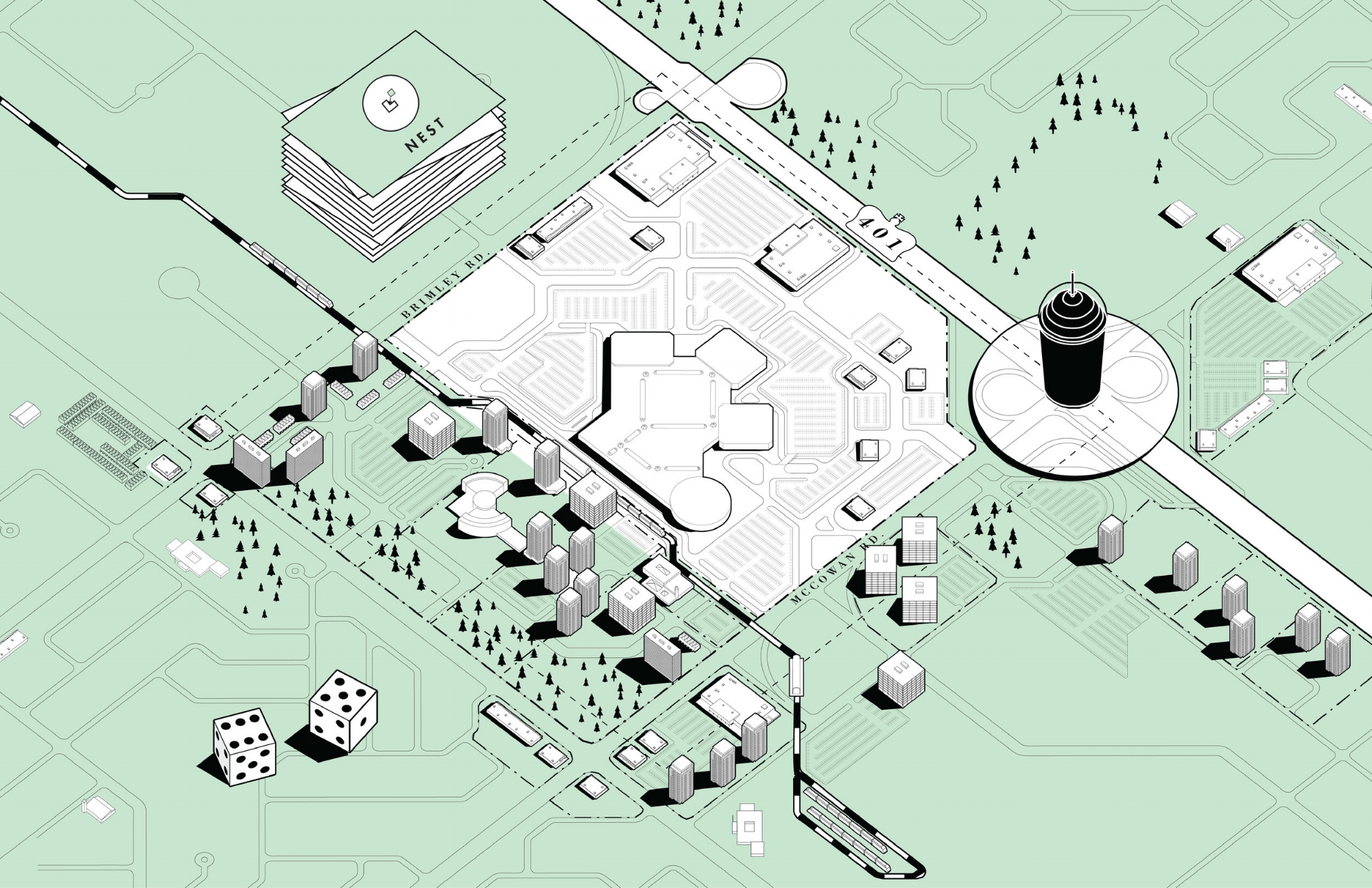The image is a detailed, rectangular sketch of a futuristic cityscape, blending elements of a circuit board and a board game. The background is primarily a light minty green, with intricate designs in white and black. On the top left, there’s a stack of large cards, with the top card displaying the word "Nest" in black font on a white-green background and a white circle above it. Surrounding this, there's a detailed, modern urban scene with skyscrapers, trees, and roads, leading into the central area that resembles a major shopping mall or a city center. Diagonally extending to the right, there's a black-and-white highway. On the bottom left, there are two six-sided dice showing the number 11, with several small buildings situated just above them. Additionally, on the right side, there's a black-and-white illustration of a circle featuring what appears to be a coffee-style drink. The entire image, with its blend of cityscape and game-like elements, gives the impression of a detailed, cartoon-style map or circuit.